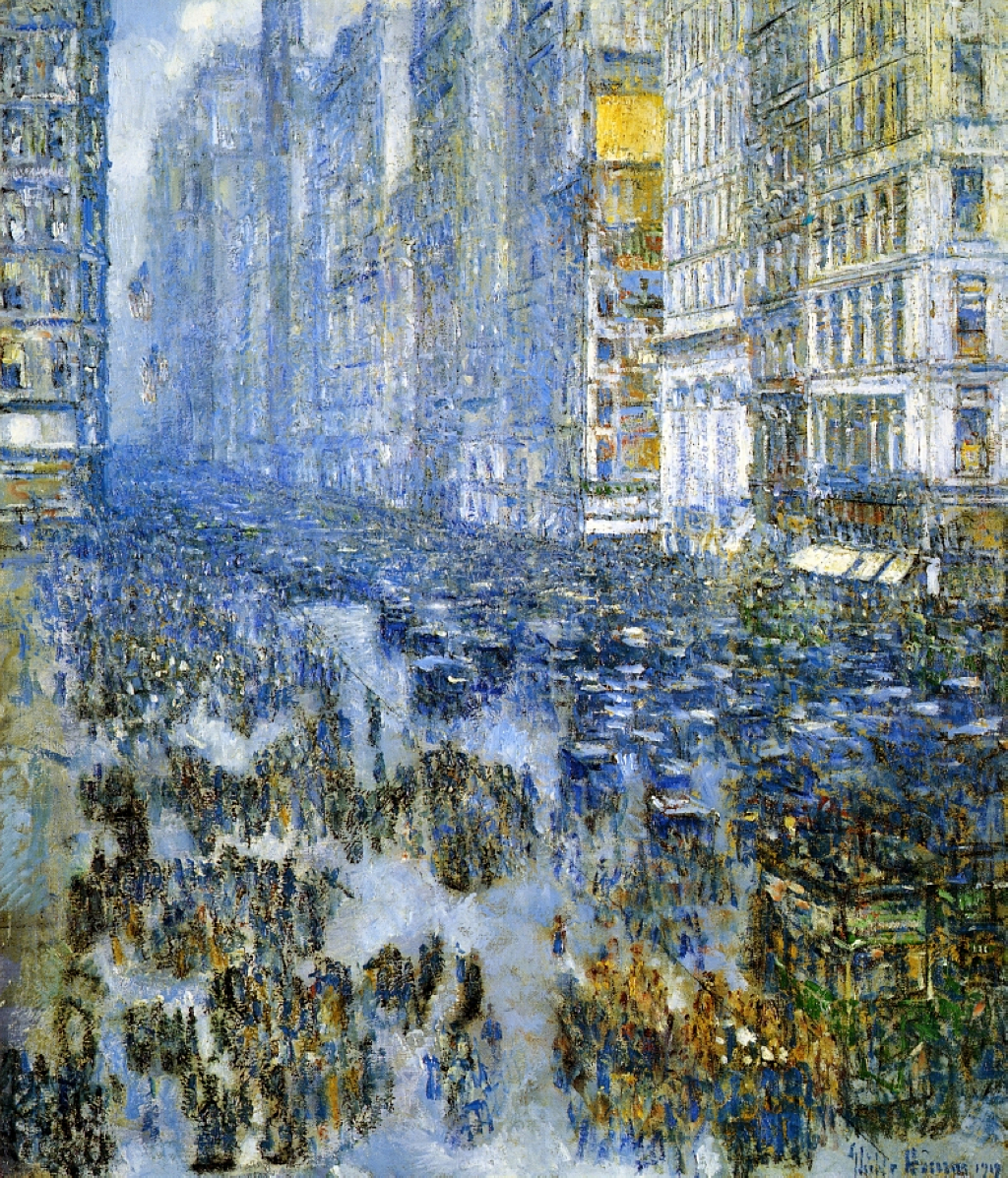This abstract painting, predominantly in blue and white hues, portrays a bustling cityscape with an impressionistic and blurry style, giving the scene a dreamlike quality. In the upper right-hand corner, tall buildings line the street, mingling shades of blue, white, and yellow. On the upper left, the side of another building can be seen, extending downwards. The middle of the street appears packed with what might be vintage cars from the 1930s, although the lack of detail makes it ambiguous. The bottom left corner features indistinct figures on a sidewalk, rendered in yellow, brown, and blue, suggesting a multitude of people. In the bottom right, an area filled with splotches of yellow and green possibly represents another structure or perhaps more people. The overall scene has a watery feel, almost as if the city were submerged, adding to the abstract and surreal nature of the artwork.